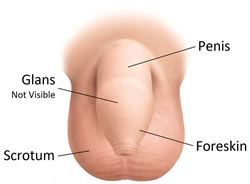The image is a detailed diagram of male genitalia, specifically a penis and scrotum, with a light tan or peach coloration indicating Caucasian skin tone. The diagram features black lines and labels pointing to key anatomical parts: the penis, foreskin, scrotum, and glands (although the glands are indicated as not visible). The illustration is presented from a frontal view, showing the penis and the wrinkled scrotum beneath it. There is no background, and the upper part of the body above the penis is either cut off or blurred. The uncircumcised nature of the penis is emphasized by the presence of the foreskin. The image appears scientific, somewhat like a medical poster, and lacks any pubic hair, adding to its clinical representation.